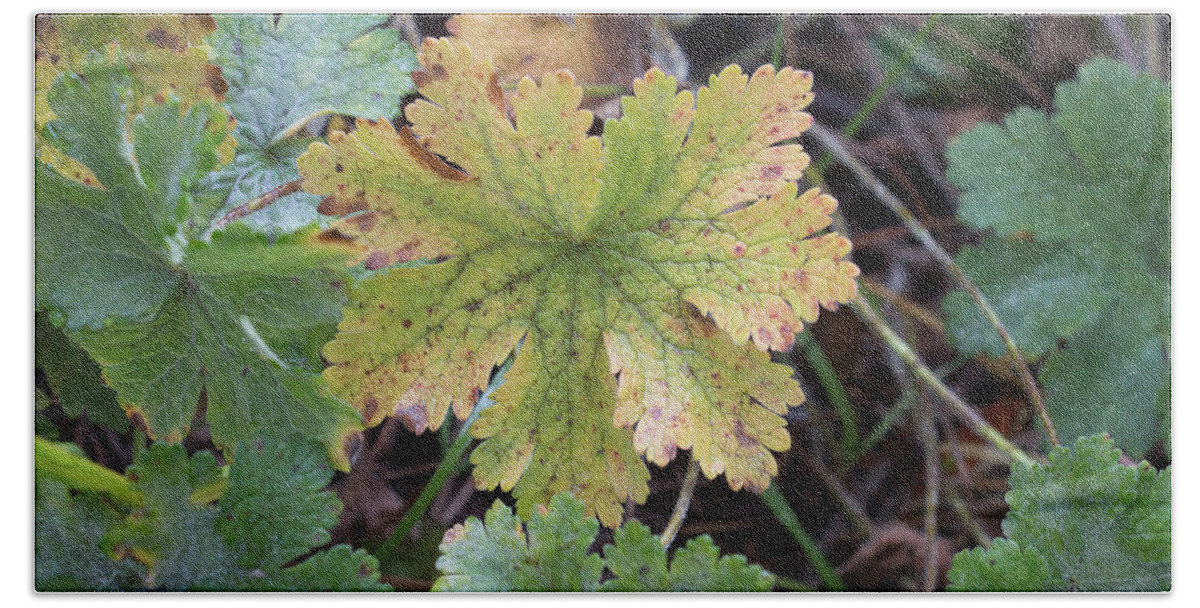The image captures a close-up of a leaf that stands out prominently against a background of numerous other leaves. The focal leaf, characterized by its green center fading to yellowish edges, displays several brown spots suggestive of deterioration akin to fall foliage as the chlorophyll diminishes. It features approximately seven to nine distinct segments or outcroppings extending from its center, giving it a somewhat textured, scalloped edge appearance. Surrounding this leaf are numerous other leaves, mostly healthier and darker green in hue, while a few also exhibit similar spots. The scene is set in a natural environment with visible brown and green stems, tree branches, and vines in the background. The ground beneath appears out of focus, but you can discern the presence of various stems weaving through the leaves, adding to the wild and natural feel of the photograph.